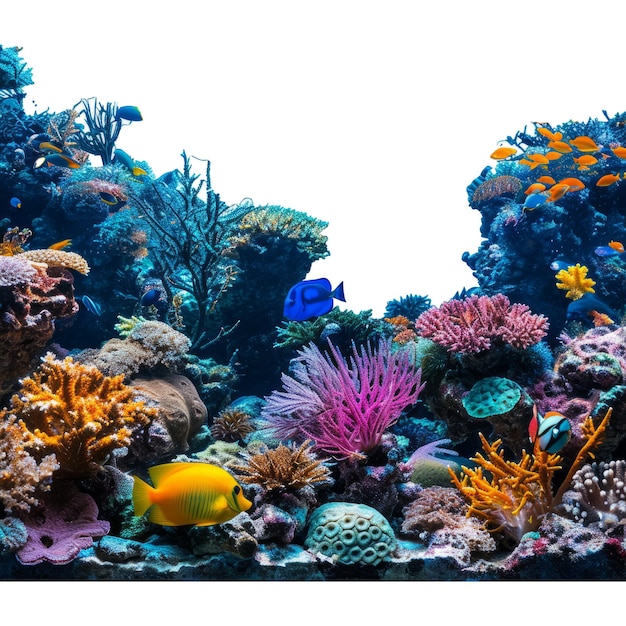The image depicts a colorful, computerized coral reef scene set against a stark white background, possibly photoshopped or brightly lit. The aquatic landscape is densely packed with various multi-colored corals and sea anemones. These include thin, mini-branched corals in purplish pink, squatter multi-branched corals with white and orange coloration, and dark blue, rock-like corals resembling human brains. Wispy-armed corals flow amidst the detailed underwater flora.

Interspersed within the vibrant coral are various fish: a bright yellow fish in the foreground, a vivid blue fish swimming slightly further back, and a small school of about a dozen orange fish in the upper right. A distinctive small white and black striped fish with orange fins is also present. The overall palette blends hues of yellow, pink, lavender, light aqua, black, orange, and green, creating a visually rich and dynamic underwater tableau. Despite the detailed portrayal of marine life, the image curiously lacks any direct indication of water, emphasizing the fish and corals against an immaculate white backdrop.